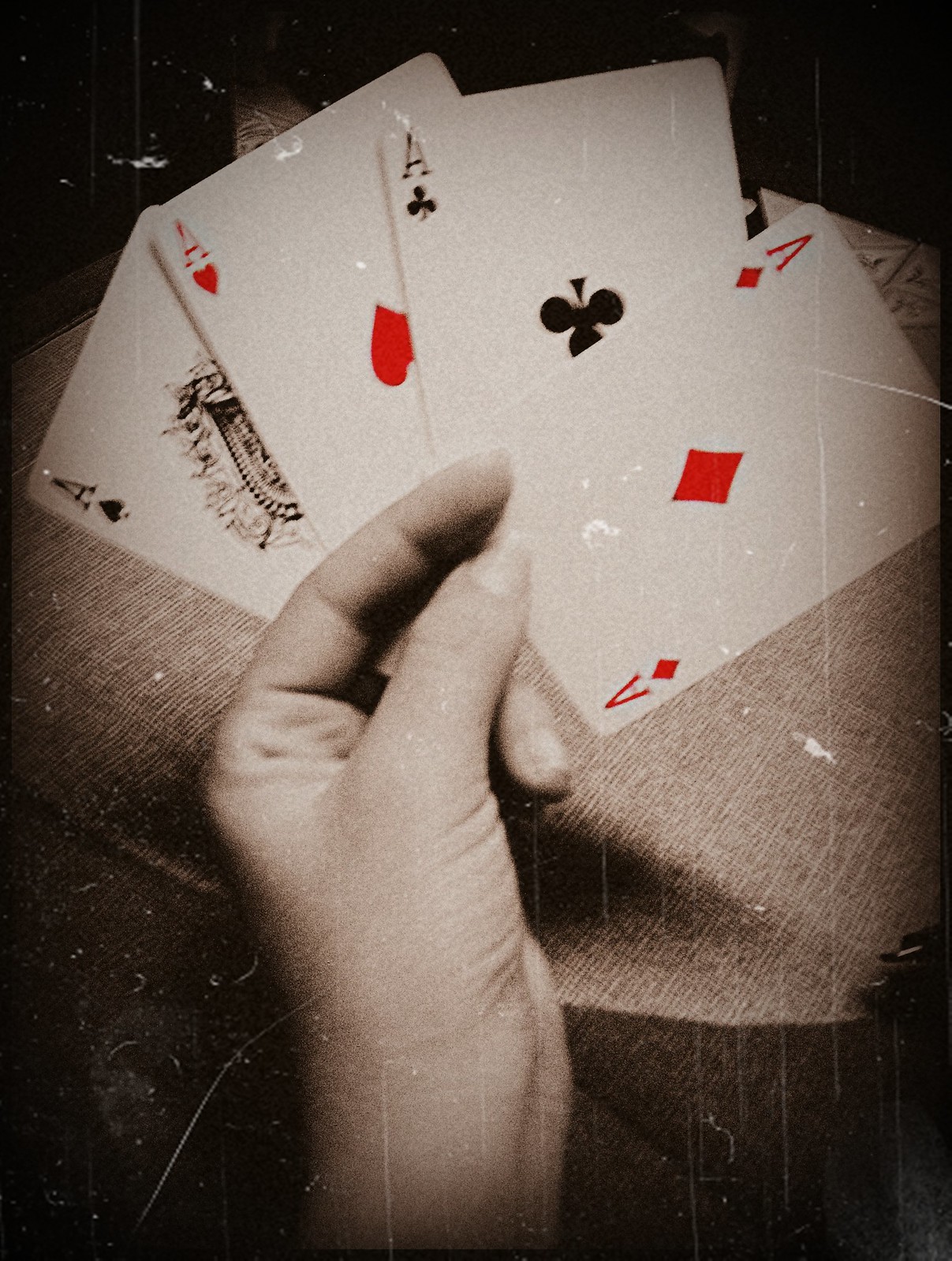The image is a stylized, sepia-toned photograph reminiscent of early 1900s photography, complete with cracks and scuff marks that evoke the aged appearance of old film. The primary focus of the image is an elegantly pale left hand with long fingernails, suggesting it belongs to a woman. Her hand rests atop a table draped in potato sack cloth, and she appears to be holding four playing cards. The cards, strikingly vibrant in contrast to the rest of the image, are the four aces: hearts, diamonds, clubs, and spades, all from a standard deck. The cards appear pristine and digitally enhanced, possibly even inserted, as they differ markedly from the worn texture of the rest of the scene. Due to the unnatural positioning of the woman’s fingers, which do not convincingly grasp the cards, the image likely is an AI-generated artwork.